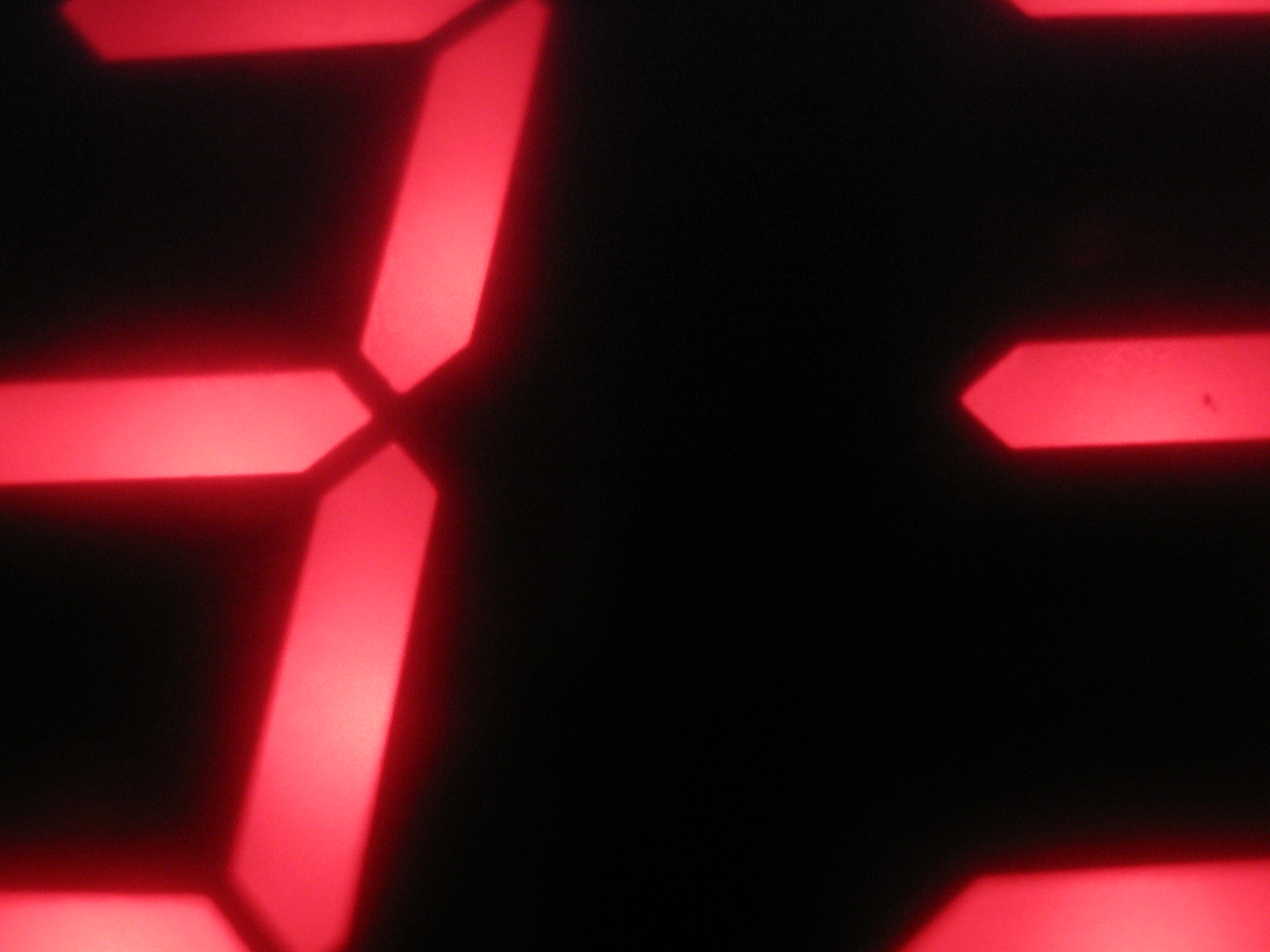A close-up image of a digital clock display, focusing on the minute segment which prominently shows the number "33." The digits are brightly illuminated, making them stand out against the dark background of the clock's face. The photograph captures the sleek, modern design of the timepiece with crisp clarity, emphasizing the precision of the timekeeping device.